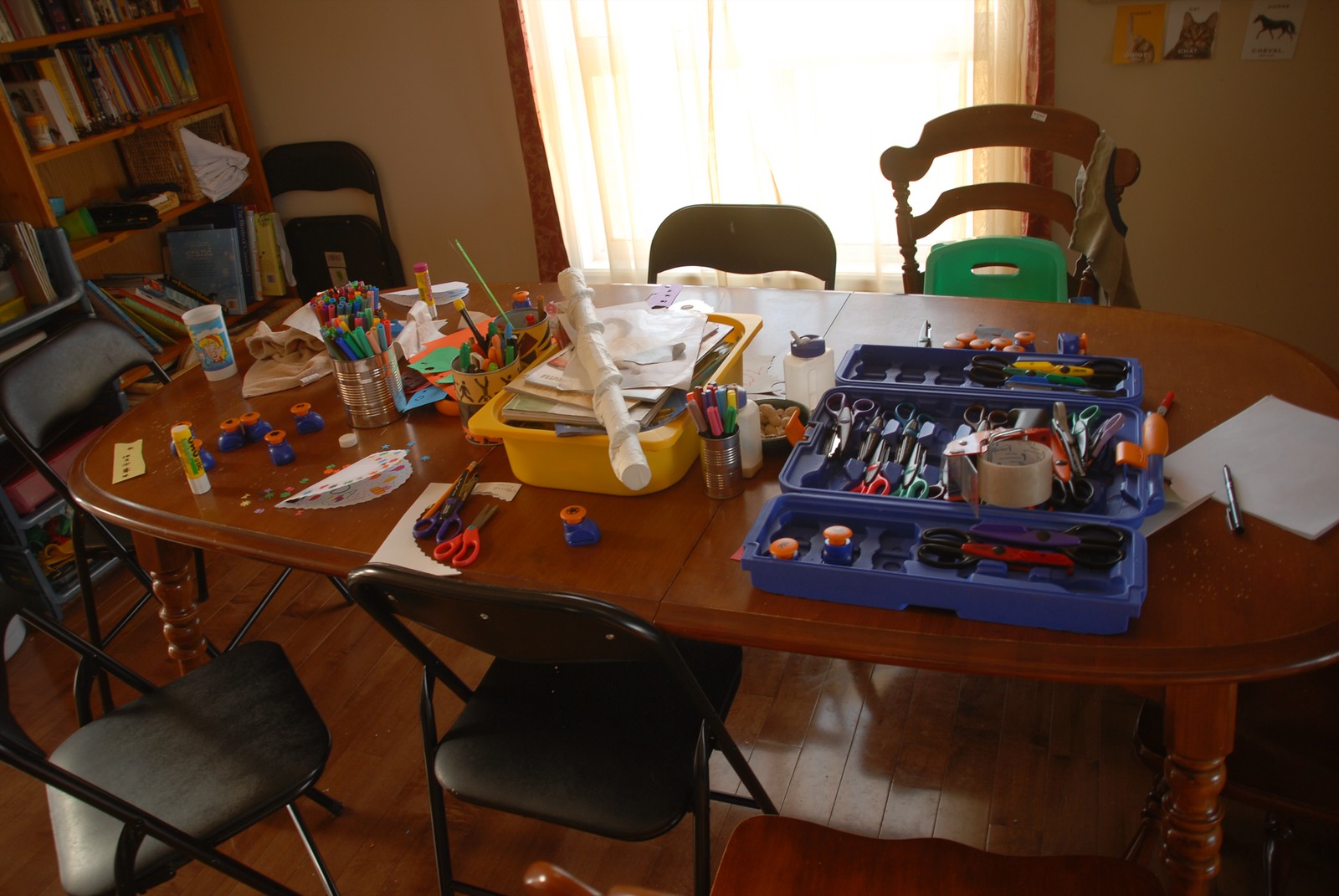The image depicts a spacious dining room repurposed as an art space, characterized by beige walls complemented with wooden trim. The room features a darker wooden floor and is anchored by a large brown wooden table cluttered with various art supplies. Around the table, there are six seats in total, with five fully visible and one partially visible in the bottom right hand corner. The table itself is strewn with creative materials, including a prominent blue art box, a yellow bin filled with papers and construction supplies, scissors, markers, cups, and numerous other items ideal for crafting.

In the background, a bookshelf brimming with books and assorted objects can be seen, with a chair stacked behind it. One of the chairs in the background holds a blue booster seat and an apron, suggesting activities geared towards young children. The room also features a window adorned with a sheer curtain bordered in red, and nearby, several pictures are tacked up on the wall, adding color and inspiration to the creative atmosphere.